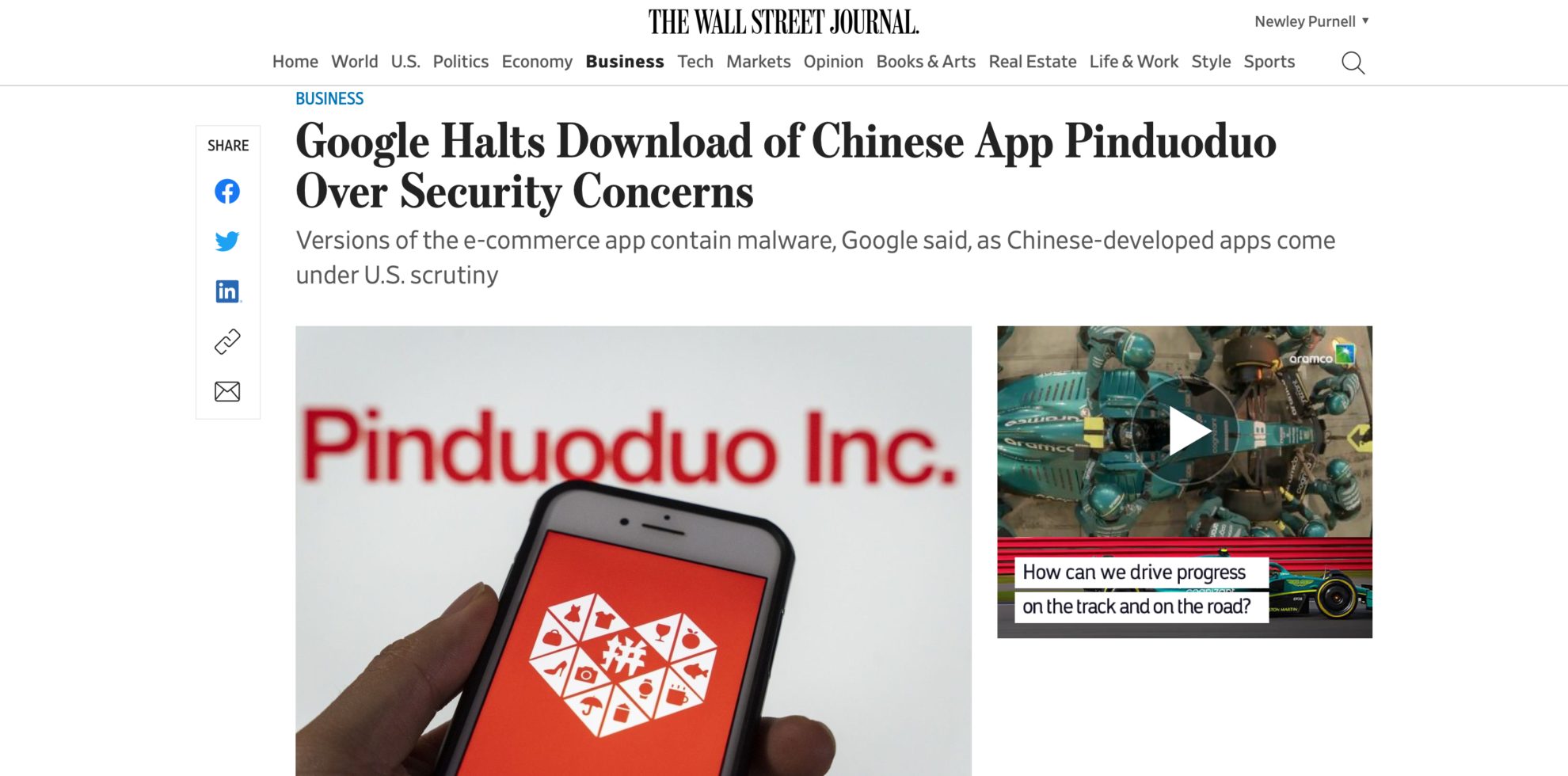The image appears to be a screenshot of The Wall Street Journal's website, featuring a clean white background. At the top center, "The Wall Street Journal" is prominently displayed in bold black text. Directly below this title, there are several navigation tabs including "Home," "World," "U.S.," "Politics," "Economy," "Business," "Tech," "Markets," "Opinion," "Books and Arts," "Real Estate," "Life and Work," "Style," and "Sports." A search icon is located to the right of these tabs.

The "Business" tab is highlighted in bold, indicating it has been selected. Beneath the navigation tabs, the top of the page displays the "Business" section heading in blue. Below this heading, there's a major article titled, "Google Halts Download of Chinese App Pinduoduo Over Security Concerns," written in black text. The article is supplemented with text and images underneath the headline.

On the left side of the page, there's a vertical panel featuring sharing options, allowing users to share the article via various social media platforms and email.